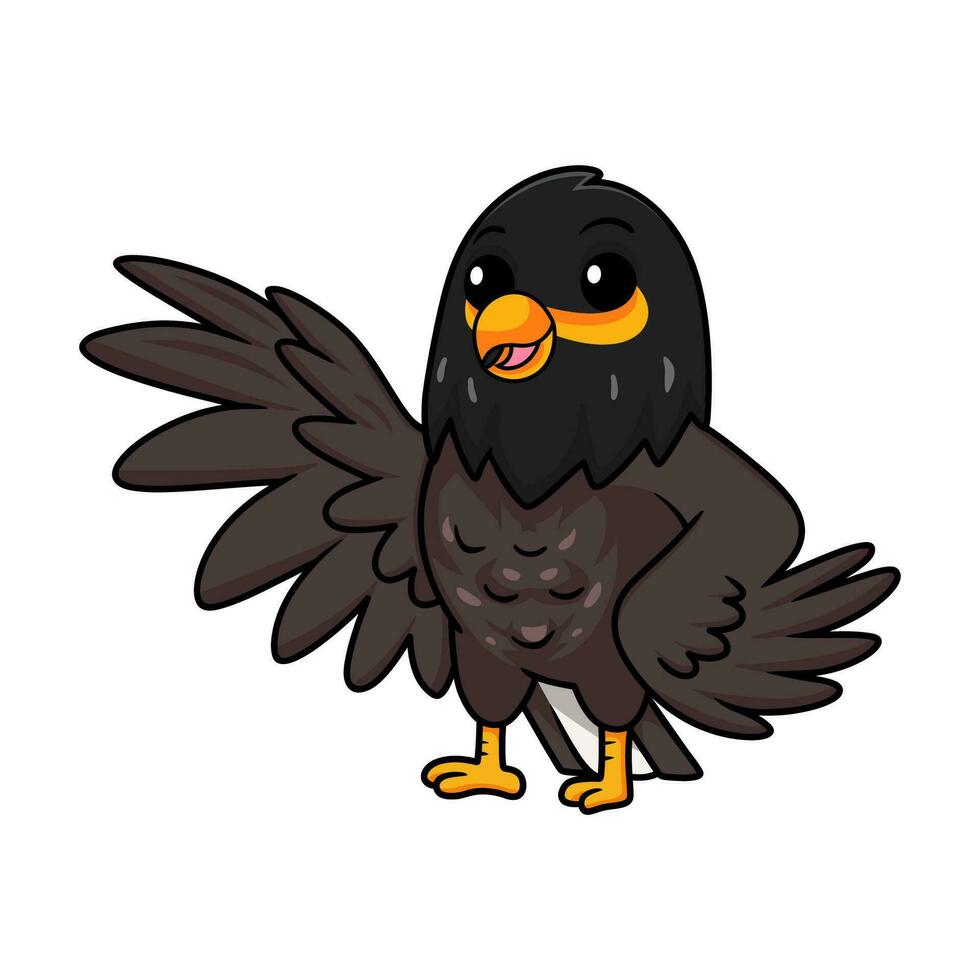This image features a hand-drawn cartoon character of a slightly sassy-looking eagle standing against a solid white background. The eagle has a black head with subtle curved lines for eyebrows and large white eyes, each containing tiny black circles with small white centers. Below its eyes are wide orange and yellow stripes. The bird's short, squat beak, colored in bright orange and yellow, is open to reveal a small pink tongue, making it appear as if the eagle is smiling. The body of the eagle is primarily charcoal gray with various shades of gray on its chest and some light purplish-gray streaks on its underside. The wings are notably large for the size of the bird, with the right wing extended outward and the left wing bent at the elbow, resting on its hip. The tail features a mix of gray and white feathers, with the underside being white. Completing the look are the bird's two small orange feet, neatly outlined in black.